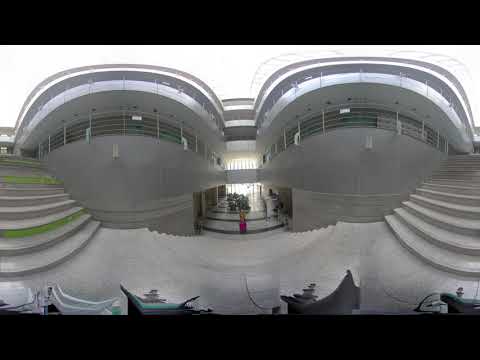This low-resolution, warped, panoramic photograph or photorealistic image presents a wide and expansive view of an architectural complex. The image, bordered by thick black rectangles at the top and bottom, includes a central staircase made of white stone or concrete, descending away from the viewer and leading to a striped black and white floor. The left and right sides of the image feature gray cement staircases, with the left showing occasional patches of green, possibly grass or paint. Towering above the viewer on each side are identical multi-story gray buildings with long balconies and curved corners. These buildings seem to converge towards the back of the image, forming a continuous structure. There are multiple levels and connecting bridges between them. At the bottom of the central staircase, a pink object stands out against the otherwise muted tones. The background above the complex is white, enhancing the contrast and adding to the surreal feel of the image.